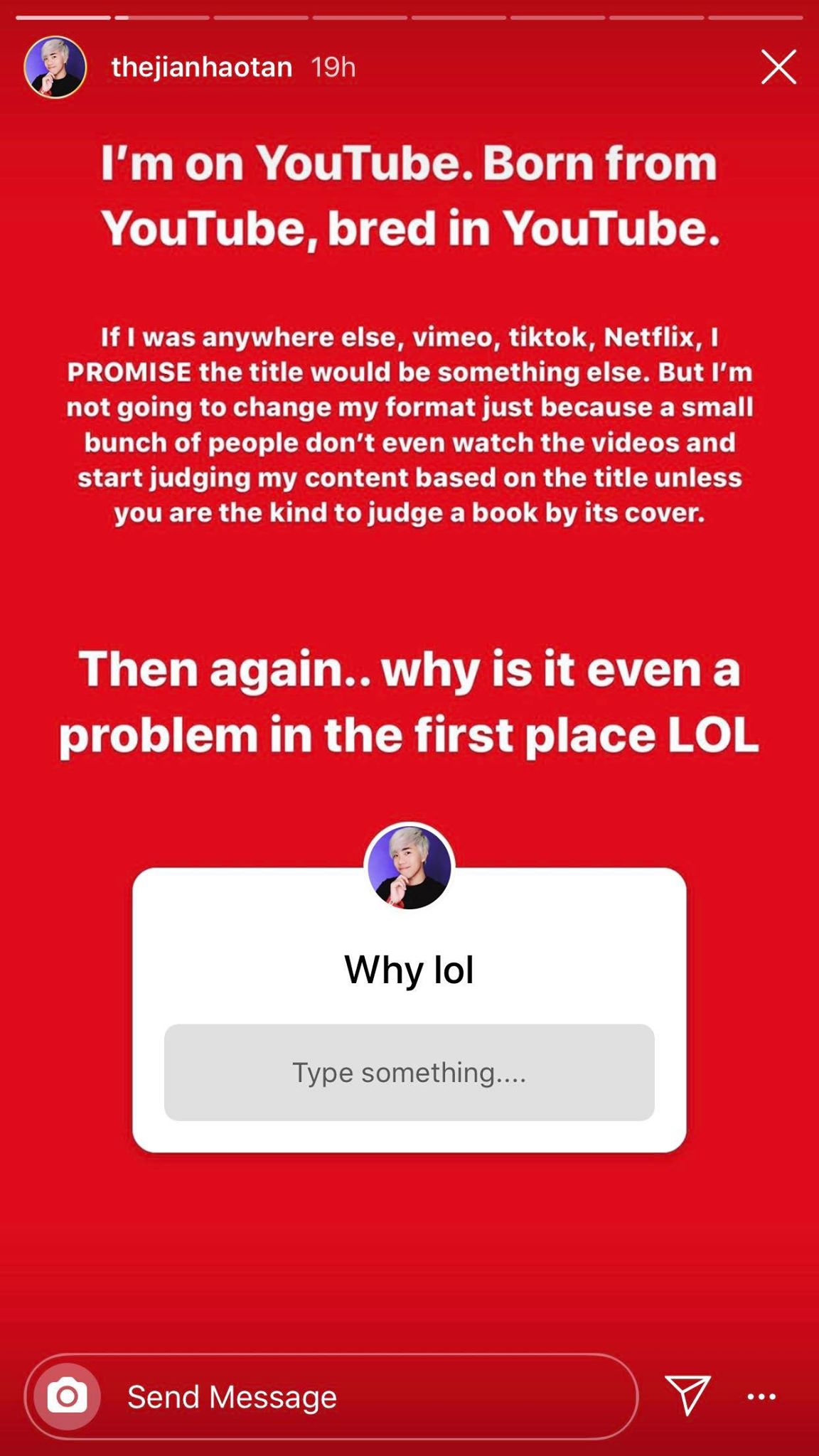In the upper left corner of the image, there is a small circular inset featuring a person with blonde hair wearing a black t-shirt. Next to the circle is the screen name "JIANHAOTAN" in bold white text, followed by "posted 19 hours ago." Below this, a text reads: "I'm on YouTube, born from YouTube, bred in YouTube. If I was anywhere else, Vimeo, TikTok, Netflix, I PROMISE the title would be different. But I'm not going to change my format just because a small bunch of people don't watch the videos and start judging my content based on the title. Unless you judge a book by its cover."

Further down, the text continues with: "Why is it even a problem in the first place? LOL." The "LOL" is emphasized in all capital letters.

Below this text, the screen name "JIANHAOTAN" appears again. Underneath, in black text, it reads "YLOL," and there is an open text box with a light gray background prompting "type something..." followed by ellipses. At the bottom of the image, there is a large search bar with an option to "send message" next to a small white camera icon inside a circle.